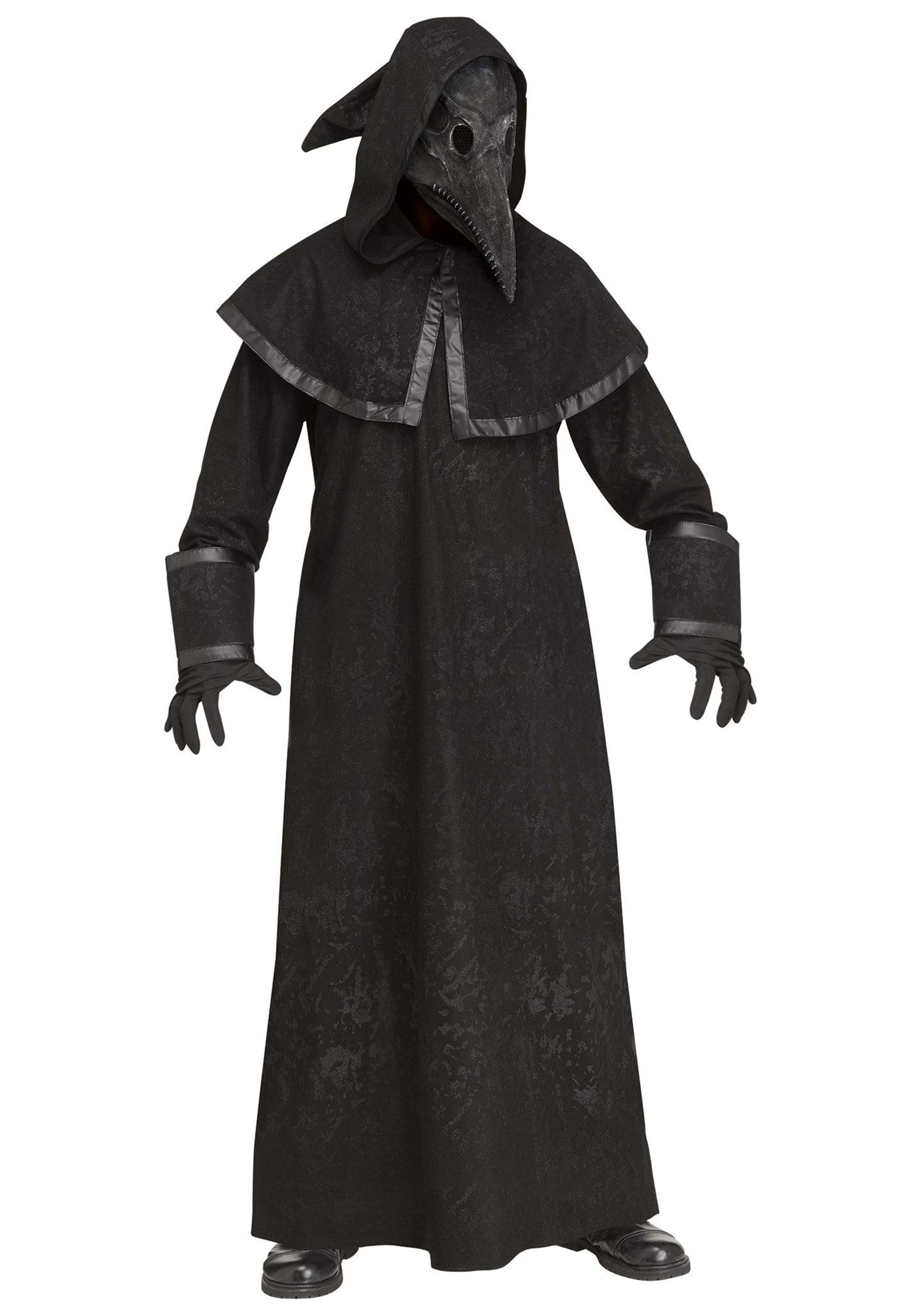This image features a person dressed in a detailed plague doctor costume, presented against a pure white background. The individual is clad in a long black robe or tunic that extends to their feet, with a black capelet draped over their shoulders. The outfit includes black boots and thick black gauntlets with large cuffs and a vinyl-like border that matches the edges of the capelet. Their hands are covered in black gloves. A black hood obscures their head, and their face is hidden behind a black mask designed to resemble a bird's skull, complete with a long, narrow, pointy beak and dark eye holes. Intricate details like staple marks along the beak add to the eerie, death-like appearance of the ensemble. The overall look evokes a mixture of a historical plague doctor and a character from a dark fantasy or horror setting, reminiscent of costumes seen in video games like Assassin's Creed or Saw.